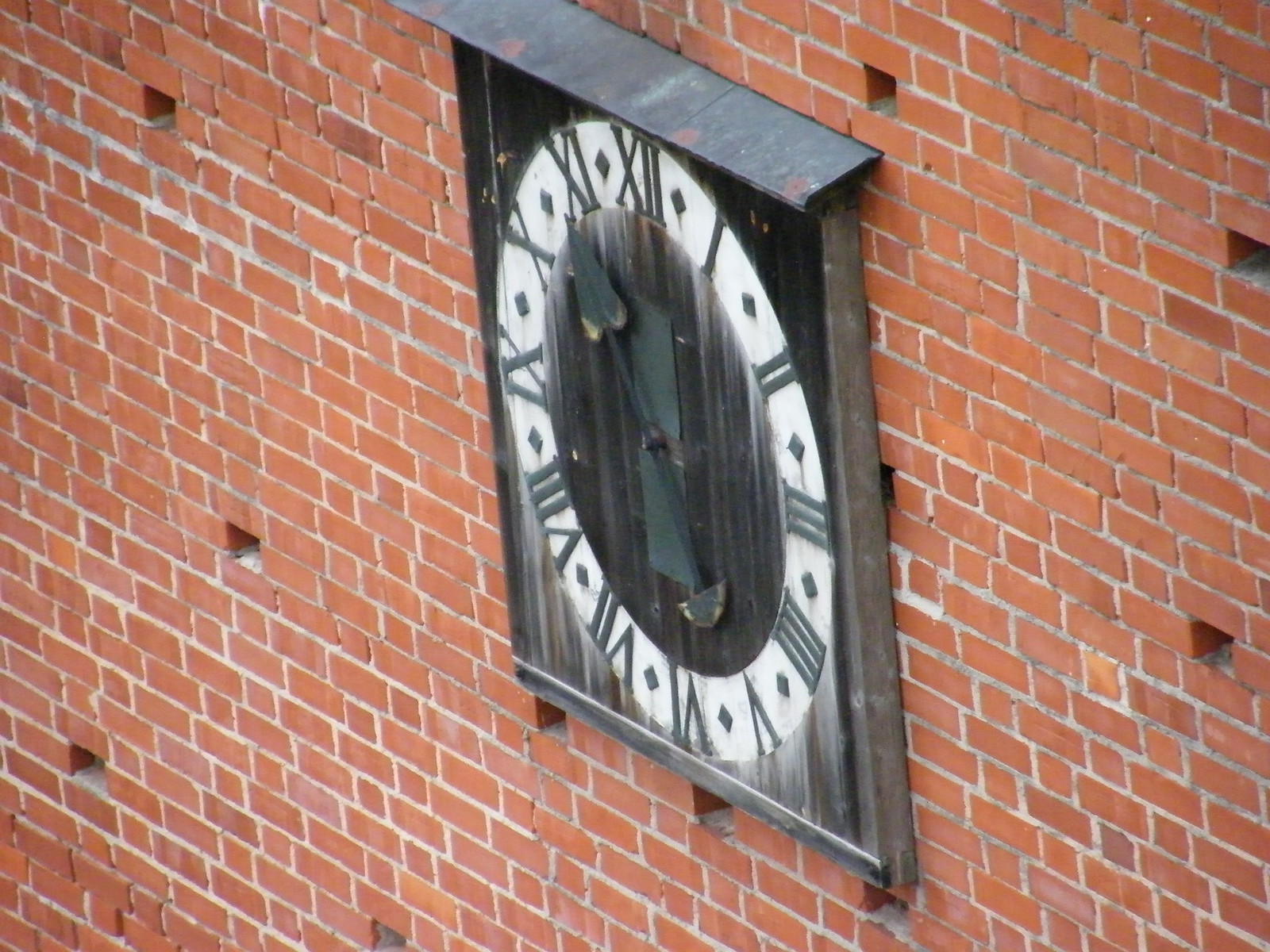The image depicts a large clock mounted on a diagonally-patterned red brick wall, which has evenly spaced holes where some bricks are missing. The brick wall could be either an exterior or an interior surface as there's no background visible. The clock itself is encased in an old, possibly rusted, black metal frame that is square, though the clock face is round. The clock displays black Roman numerals set against an aged, white background that appears to be fading into a central black area. The clock's hands are also black, with the time appearing to be around 11:25. The overall weathered look of both the clock and the wall suggests significant exposure to the elements.